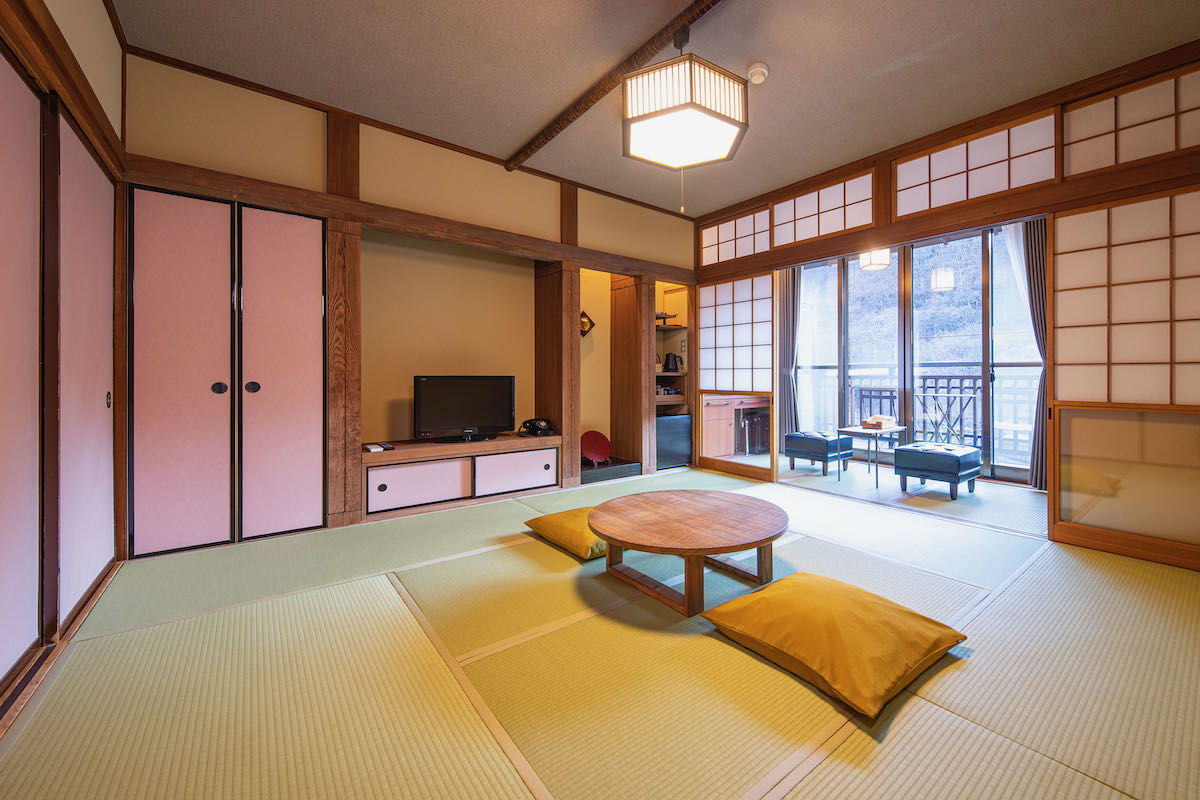The photo depicts a cozy and warm interior of a living room or perhaps a studio room with a noticeable Japanese style influence, given its minimalist decor and inviting, floor-seating arrangement. Dominating the room is a large-screen TV neatly placed inside an entertainment center with storage drawers below. Adjacent to this are two sets of white closet doors, which add to the room's storage solutions.

Central to the room's design is a round, low-height table suited for sitting around in a cross-legged manner, accompanied by two large yellow pillows positioned on either side, inviting guests to sit and gather. The floor is adorned with large carpet squares, adding a textured, soft feel to the space.

Wooden elements frame the room, highlighted by several beams crossing the ceiling. Suspended from the central beam is a distinctive large light fixture shaped like a hexagonal lantern, possibly with a pull cord, casting a soft glow over the circular table below. The presence of another smaller light next to it provides additional illumination.

Adding to the ambiance, the room features a door wall that likely leads to an outdoor space, implied by the bluish tint suggesting a cold, wintry scene outside. This door wall might open to a railing, indicating a compact outside area. The overall aesthetic, enhanced by these details, presents a harmonious blend of function and serene, inviting decor.